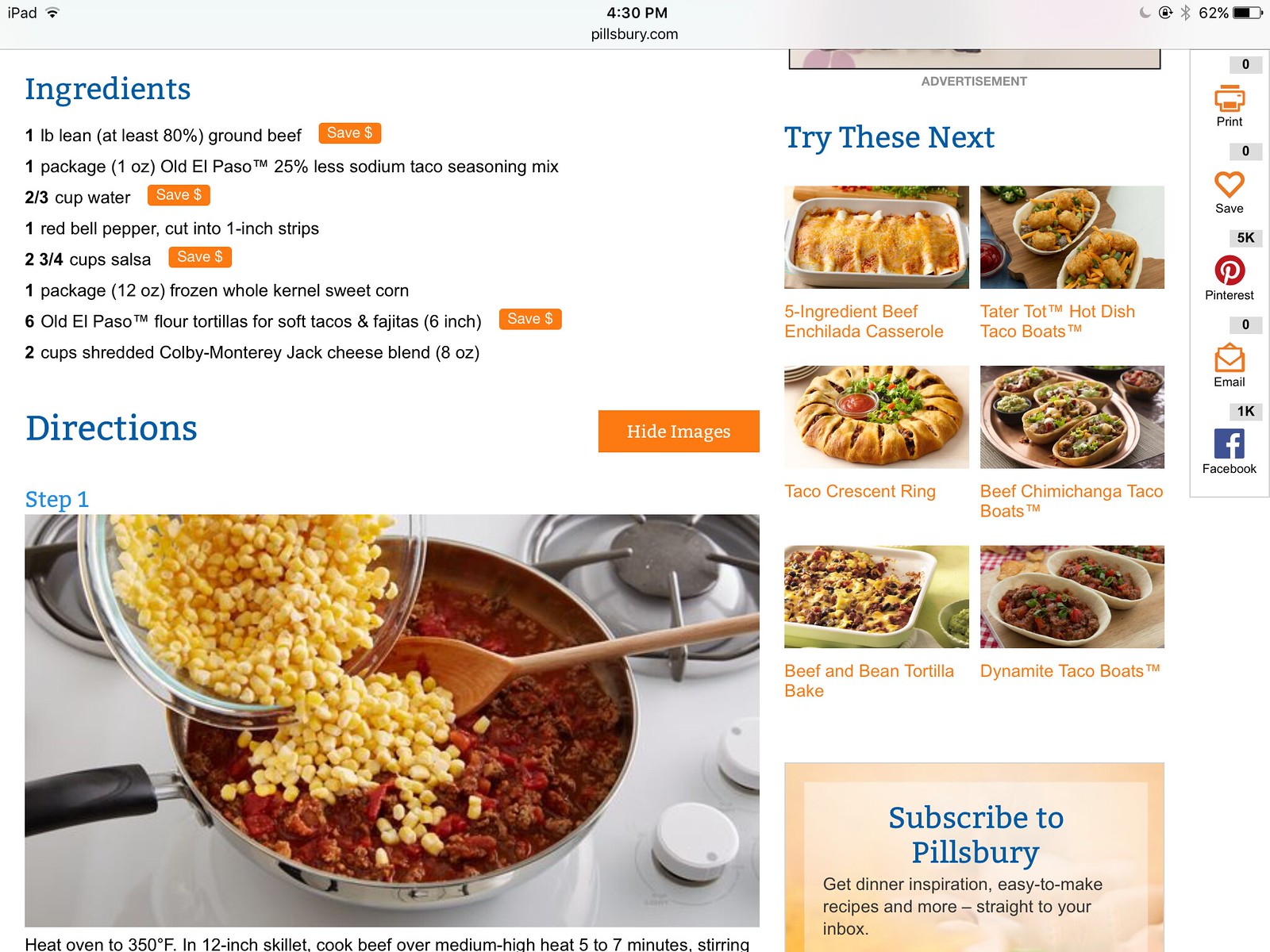This image displays a detailed recipe webpage from Pillsbury.com, viewed on an iPad. At the top, there's a blue-gray banner indicating the time as 4:30 PM, a Wi-Fi symbol, and the battery level at 62%. “iPad” is noted in the upper left corner. Directly below, the Pillsbury.com site name is prominently featured. 

The main portion of the page is centered around a recipe with a white background printed in blue and black text, listing the following ingredients:

- 1 pound lean (at least 8%) ground beef
- 1 package (1 ounce) Old El Paso™ 25% less sodium taco seasoning mix
- 2/3 cup water
- 1 red bell pepper, cut into 1-inch strips
- 2 3/4 cups salsa
- 1 package (12 ounces) frozen whole kernel street corn
- 6 Old El Paso™ flour tortillas for soft tacos and fajitas (6 inch)
- 2 cups shredded Colby Monterey Jack cheese blend (8 ounces)

Each ingredient has an adjacent orange “Save” button, some with a dollar sign symbol, indicating potential savings. 

Below the ingredients list, "Directions" appears in large blue text. Step 1 is accompanied by an image of someone pouring corn into a pan with red sauce on a stove, and the instructions read: "Heat oven to 350 degrees Fahrenheit. In a 12-inch skillet, cook beef over medium heat for 5 to 7 minutes, stirring."

On the right side of the page, there's a section called "Try These Next" with pictures of six other dishes, inviting users to explore additional recipes. At the very bottom of the page, there’s an option to subscribe to Pillsbury updates. The overall layout is clean, showcasing a mixture of text and images designed to guide users through the recipe seamlessly.